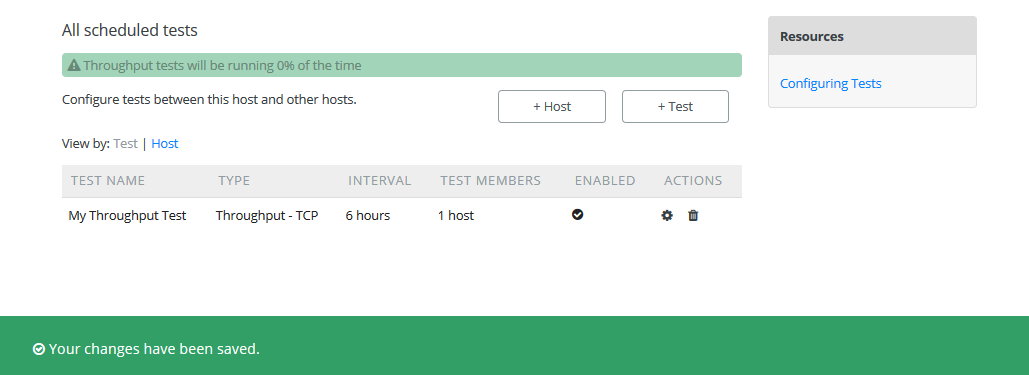In the image, we have a detailed screenshot of a test website interface. On the far left side, there is a sidebar listing all scheduled tests in text format. Below this section, a green title bar displays a warning icon – a black triangle with a lowercase letter 'i' inside it – accompanied by the text, "The throughput test will be running 0% of the time."

To the far right of the interface, there is a rectangular block labeled "Resources." Directly below this block, there is a "Configuring Test" button.

Returning to the left side of the interface, there is a section detailing configured tests between hosts. Adjacent to this section on the right are the "Host" and "Test" buttons. Below this row, the interface provides an option to view tests by categories with a "View By" dropdown, followed by a small vertical line separator, and a "Host" button highlighted in blue.

Beneath these sections, there is a gray rectangle displaying column headers for a test table. The headers include: Test Name, Type, Interval, Test Member, Enabled, and Actions. Under this table section, a specific test named "My Throughput Test" is listed. Its details are as follows: 
- Type: Throughput-TCP (capitalized)
- Interval: 6 hours
- Test Members: 1 host
- Enabled: Indicated with a question mark enclosed in a black circle
- Actions: Settings icon and a garbage icon for deletion